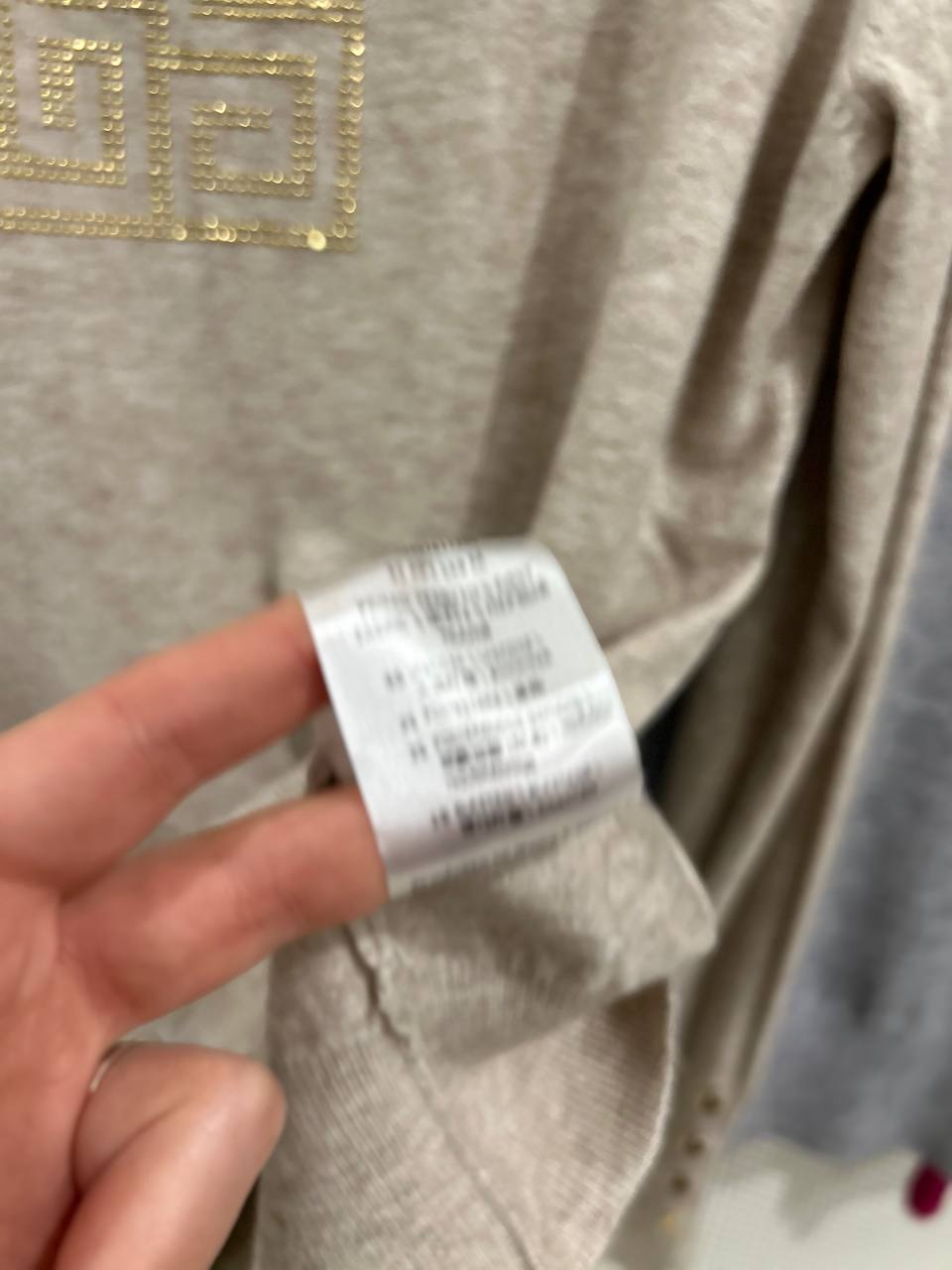This is a color photograph featuring a close-up view of a clothing label held by a person's fingers. The label, although not legible due to blurring, is white with black writing. The person's fingers, with medium light skin, are positioned such that two fingers are behind the label while one finger supports it from the bottom. Dominating the image is the garment itself—a grey t-shirt or top—in sharp focus. On the upper left corner of the clothing item, a gold sequin design forms a squarish coil pattern, glistening beautifully. The garment appears to have long sleeves, evidenced by what looks like three buttons at the sleeve's bottom, partially visible at the image's lower edge. In the background to the right, another grey top is slightly out of focus and appears darker in color. A small red object is situated near the bottom of this secondary garment, and the far right corner of the image shows a grey background area, adding to the overall setting.